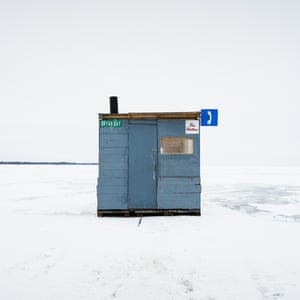In the center of the image is a small, squarish wooden shack painted light blue, situated in a vast, snowy landscape. The shack features a narrow door and a small window on the right side. The roof is brown wood, and a black cylindrical chimney extends from the top left. The roof area displays three signs: a blue square with a white telephone symbol in the top right, a white sign with red letters in the top right (illegible), and a green rectangular sign with white writing on the top left (also hard to read). The background shows a hazy, light grey sky blending with the snowy ground, and a dark green line on the horizon suggests the presence of distant trees. The monochrome sky and snow seamlessly envelop the solitary, blue shack, highlighting its isolation in the wintry expanse.